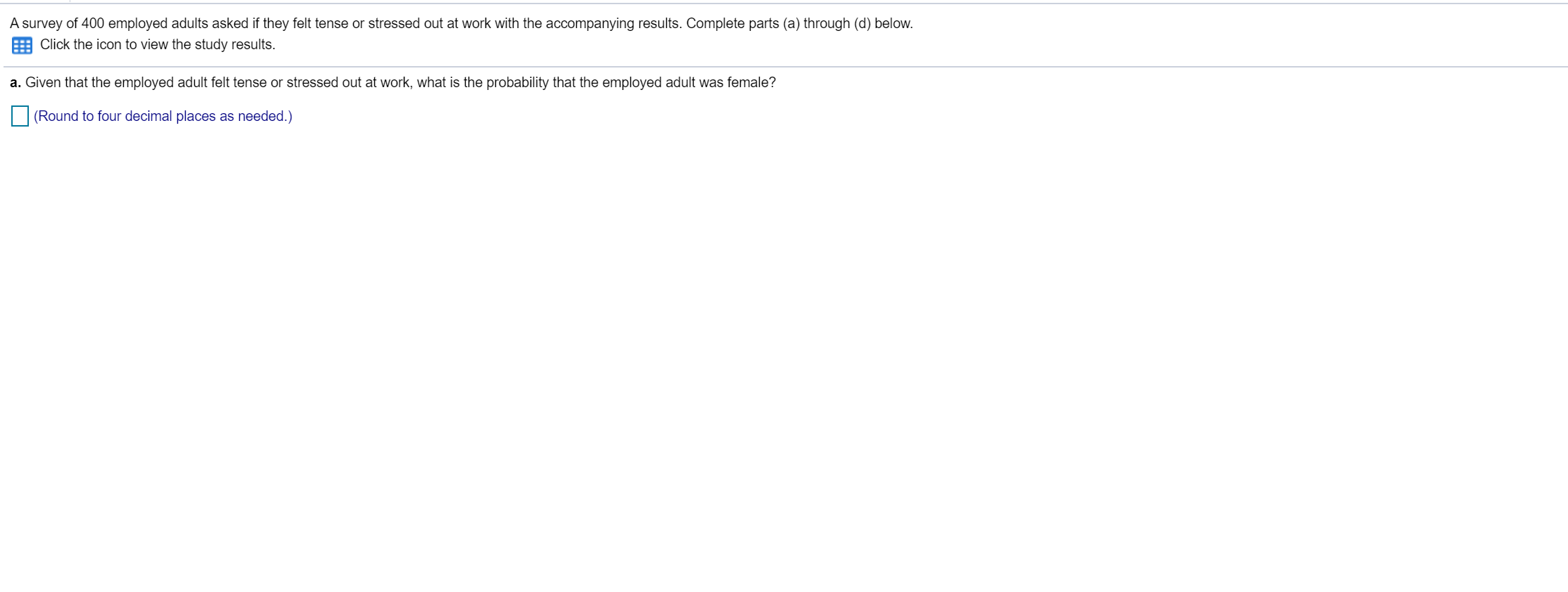In this image, a section of a page displays black text on a white background. The main content of the text details a survey of 400 employed adults, asking whether they felt tense or stressed out at work, and outlines the accompanying results. The text reads: "Complete parts A through D below." Below this statement, there is a calendar icon with an instruction to click it to view the study results.

Further down, a sub-section marked with the letter "A" asks: "Given the employed adult felt tense or stressed out at work, what is the probability that the employed adult was female?" Alongside this question is a checkbox, with an instruction to round the answer to four decimal places as needed.

Overall, the image appears to provide a snapshot of example questions and instructions from a survey or study. The layout is simple and straightforward, displaying primarily text with minimal graphical elements. The purpose seems to be to illustrate the format and type of questions in the survey.